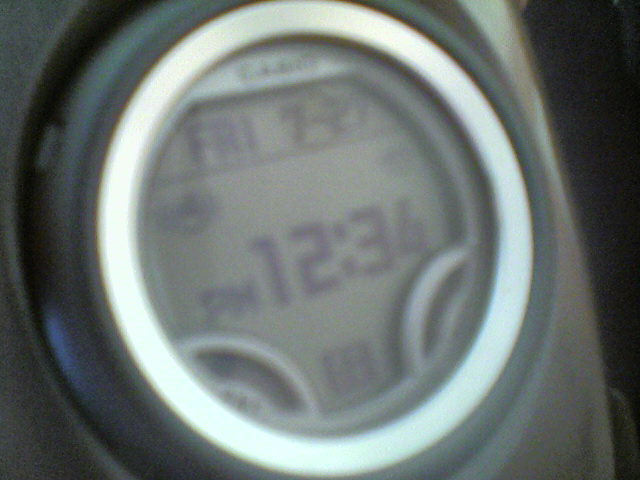The image is a very close-up, slightly blurry photograph of a digital fitness watch. The watch has a circular black face encircled first by a silver ring, then a dark grey or black bezel. The digital display shows the time as 12:34 PM prominently in the center, and above it, the day is indicated as "FRI" in all capital black letters, with the date "7-27" below it. While the display also includes additional numbers below the time, they are indistinct and possibly read "68". The surrounding background of the image appears solid black, especially pronounced in the top right-hand corner and along the right side, further emphasizing the face of the watch. The watch's structure includes a grey fascia, and though not visible, it likely has a functional and modern design akin to a sports watch or smartwatch.